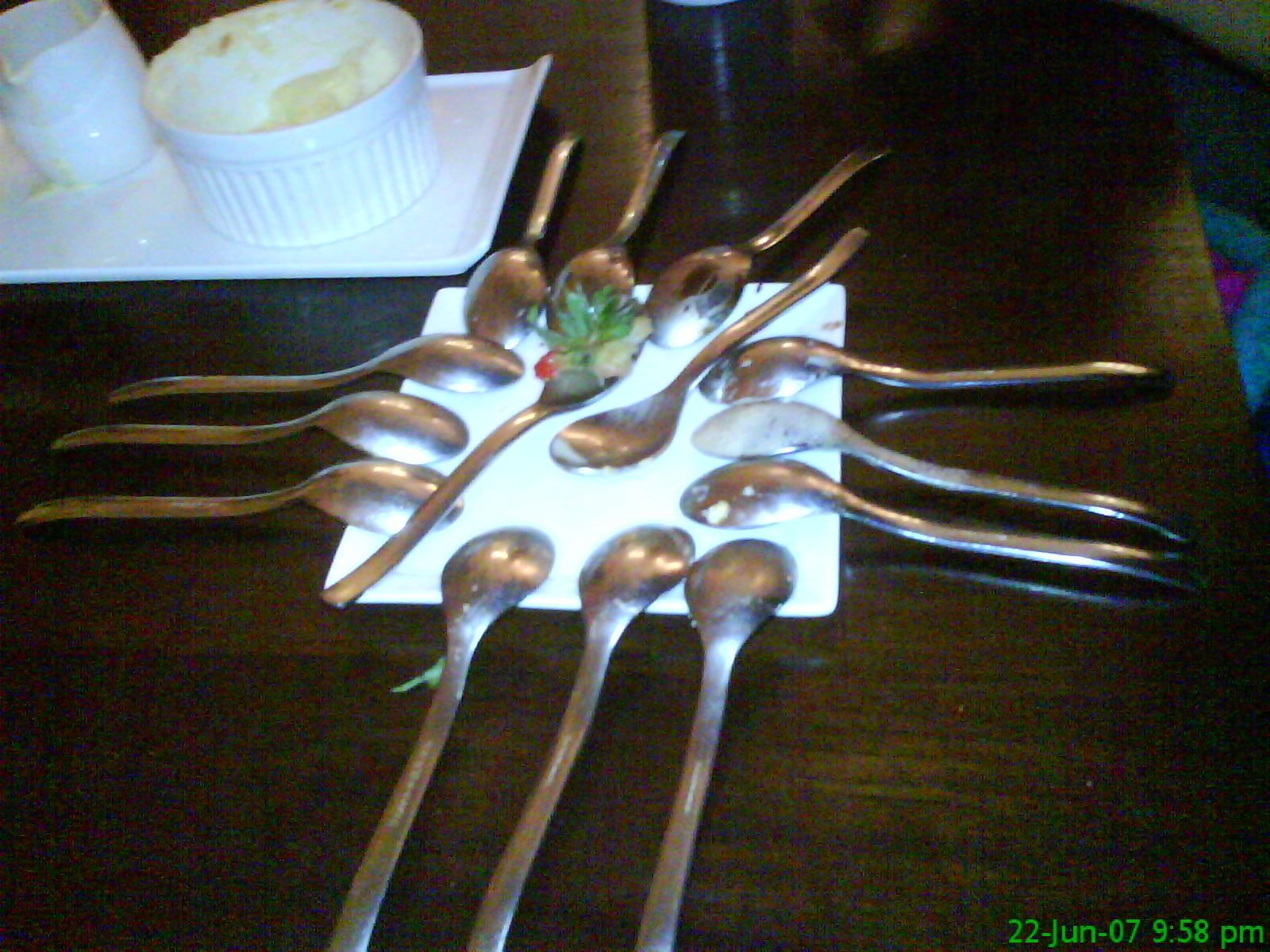The image displays a square white plate situated on a dark brown wooden table. Arranged meticulously around the plate's edges are twelve spoons, with three spoons on each side, all facing downward with their handles extending outward. In the center of the plate lie two diagonally positioned spoons facing upward, one of which holds the top of a strawberry, complete with green leaves and a hint of pinkish fruit. In the background, a white serving tray holds a white bowl, potentially filled with mashed potatoes, and a white creamer-like pitcher. The photo details are reinforced by a digital timestamp positioned in the bottom right corner, reading "22 June 07, 9:58 PM," and suggests a post-dinner scene, possibly at a restaurant, as indicated by the partially consumed food items and the overall arrangement.